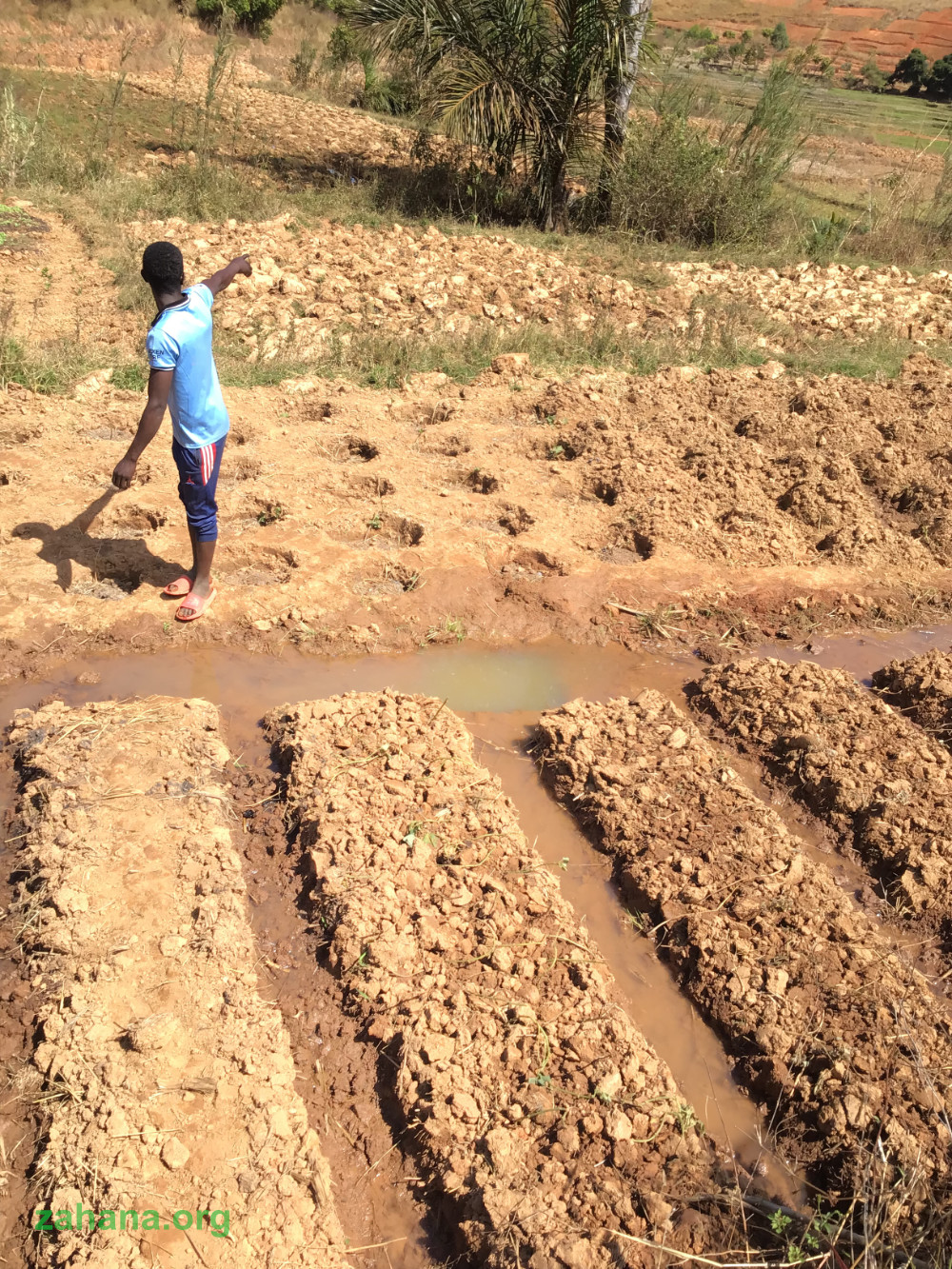In the image, a young African-American man stands in a cultivated field characterized by neatly arranged rectangular plots, likely created by hand or machine. He is situated on a slight elevation as he points towards a tree or down the hill. The scene is bathed in daylight, illuminating the predominantly light tan, muddy ground interspersed with green grass. Visible irrigation channels suggest organized planting, though the specific type of crops or trees being cultivated is unclear. The soil is marked with holes, indicating preparations for planting. The man is dressed in a light blue shirt, navy blue pants, and red sandals, drawing attention to his purposeful stance. In the background, additional trees and grassland are visible, adding depth to the landscape. The lower left corner of the image features the text "Zahana.org."